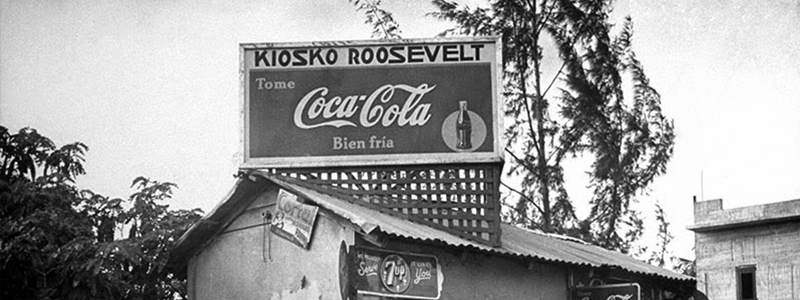This black and white photograph, taken on a clear day, captures an old rectangular building, likely from the 1930s or 1940s, with a tin metal roof. The structure appears to be a mom-and-pop store, possibly doubling as a kiosk or a small garage. The most prominent feature is a large sign fixed atop the building, held in place by a wooden framework. The sign reads "Kiosko Roosevelt" and beneath it, in Spanish, "Tome Coca-Cola Bien Fría," accompanied by an illustration of an older Coca-Cola bottle. Surrounding the building are various trees and bushes; a tall, skinny-trunked tree stands out behind it, while additional trees flank the structure on either side. In the lower right of the photo, another larger building with an entrance is partially visible.